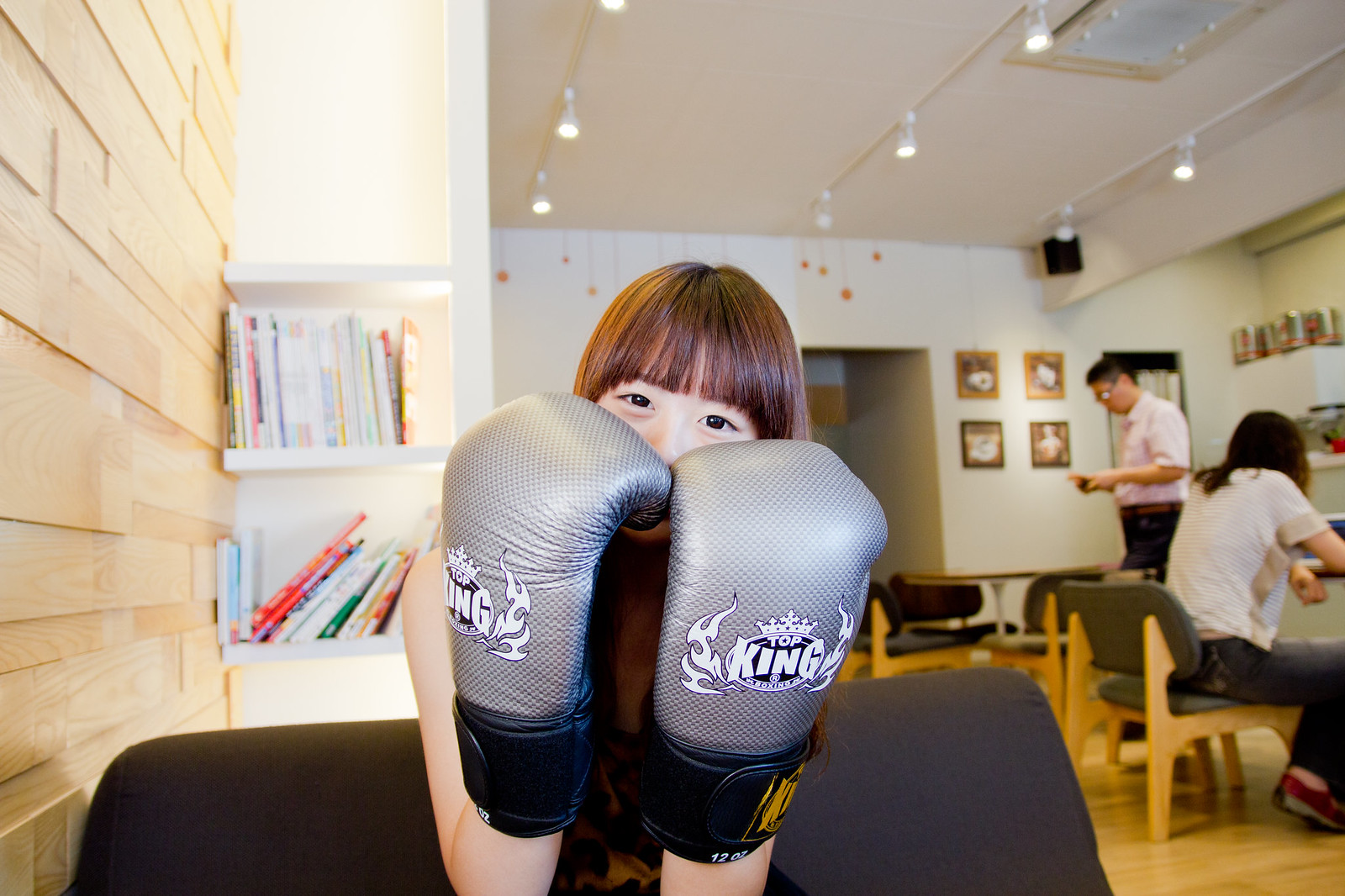This color photo captures an Asian girl around 10 years old with brown hair and bangs, inside a modern home interior. She is sitting on a low, modern wooden chair with dark cushions, leaning over the back and holding up a pair of oversized silver boxing gloves with black Velcro wrap cuffs that display a 'Top King' logo and white flame designs. Her face is mostly obscured by the gloves, but her crinkled eyes suggest she is smiling. The background reveals an open floor plan featuring light-colored wood paneling, illuminated built-in white bookshelves, and light-colored hardwood floors, possibly bamboo or laminate. Track lighting arrays accentuate the ceiling, and artworks decorate the walls. To the right, an older man who appears to be her father, dressed in a short sleeve shirt and dress pants, is sitting in a low wooden chair, looking at his cell phone, and another person with shoulder-length hair and wearing a white shirt and jeans is seated further back.